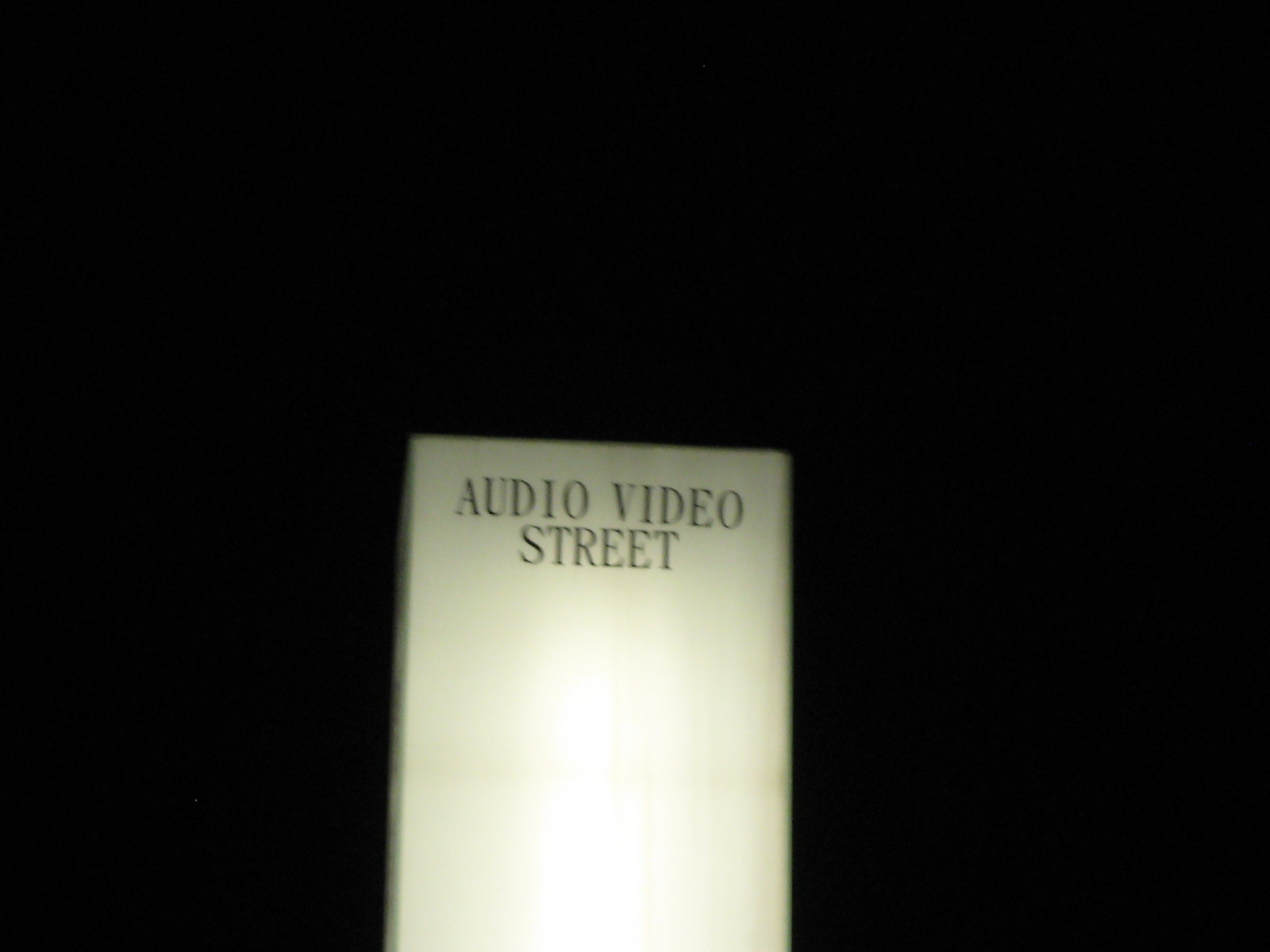The image features a completely black backdrop. In the foreground is a white rectangular object extending from the bottom and reaching halfway up the picture. At the top of this rectangle, in bold black letters, it reads "Audio Video Street," with "Audio Video" on one line and "Street" centered beneath. The rectangle has a barely discernible grayish border around it. The brightest part of the rectangle is at the center, seemingly illuminated by a flash, creating a glowing effect that makes this section appear almost as if reflecting light. The rest of the image outside this rectangle is pitch black and lacks any visible detail or context, adding to the overall mystery of the scene. The edges of the rectangle appear blurred, possibly due to out-of-focus capturing or the nighttime setting.